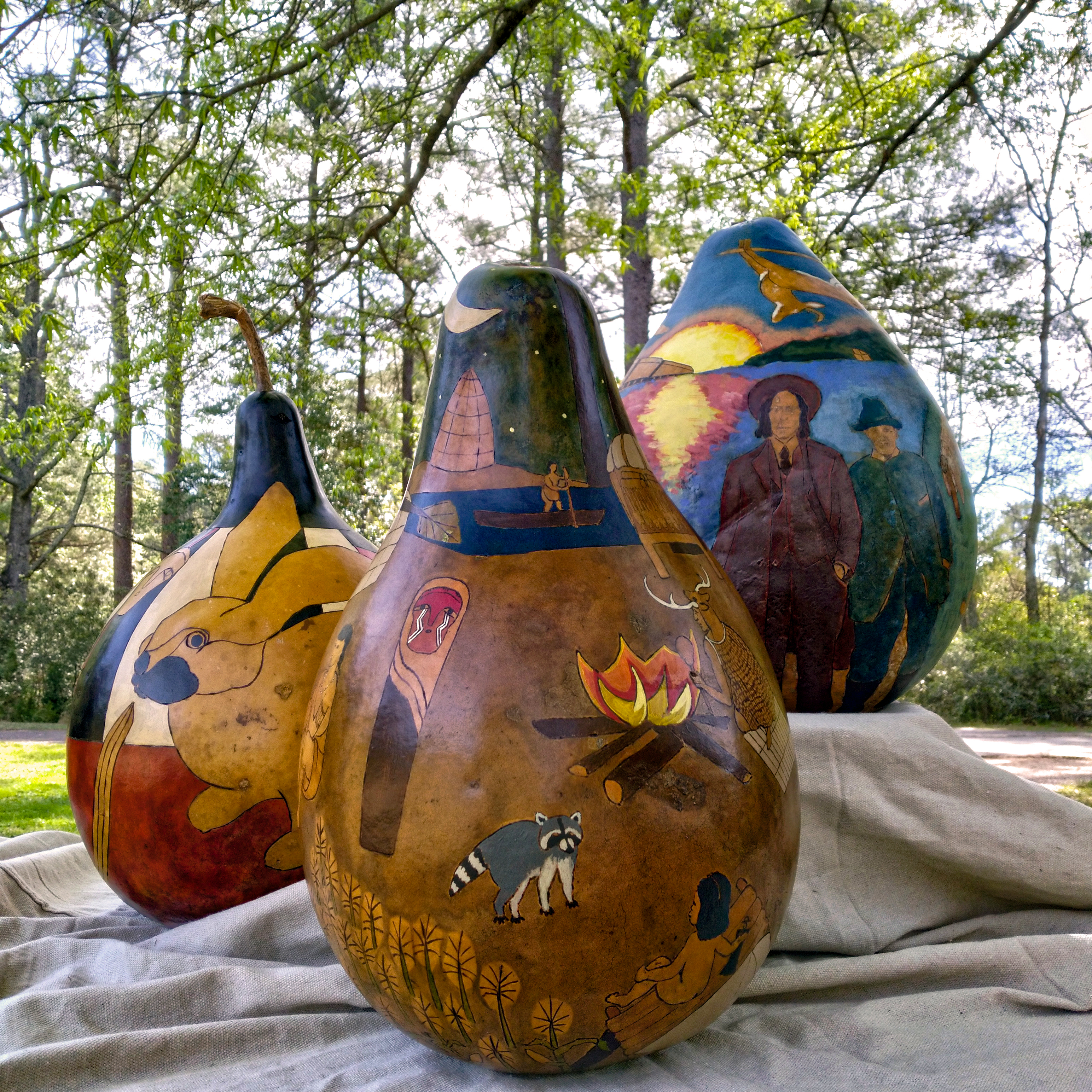This photograph showcases three artistically decorated, pear-shaped gourds placed on a white cloth, serving as a protective drop cloth, atop a table. The backdrop features a serene forest with thin, tall trees adorned with green foliage. The central gourd, painted brown, vividly depicts a raccoon and a campfire, surrounded by trees, people, and other elements like a crying totem pole and a naked figure in a river guiding a log with a stick. The gourd on the left is adorned with a yellow rabbit, accented by blue and red hues. The gourd on the right, predominantly blue, portrays two individuals dressed in red and green suits with matching hats, standing near a horse with a setting sun in the background. All these intricate details suggest the work of a skilled artist, making each gourd a unique piece of art.